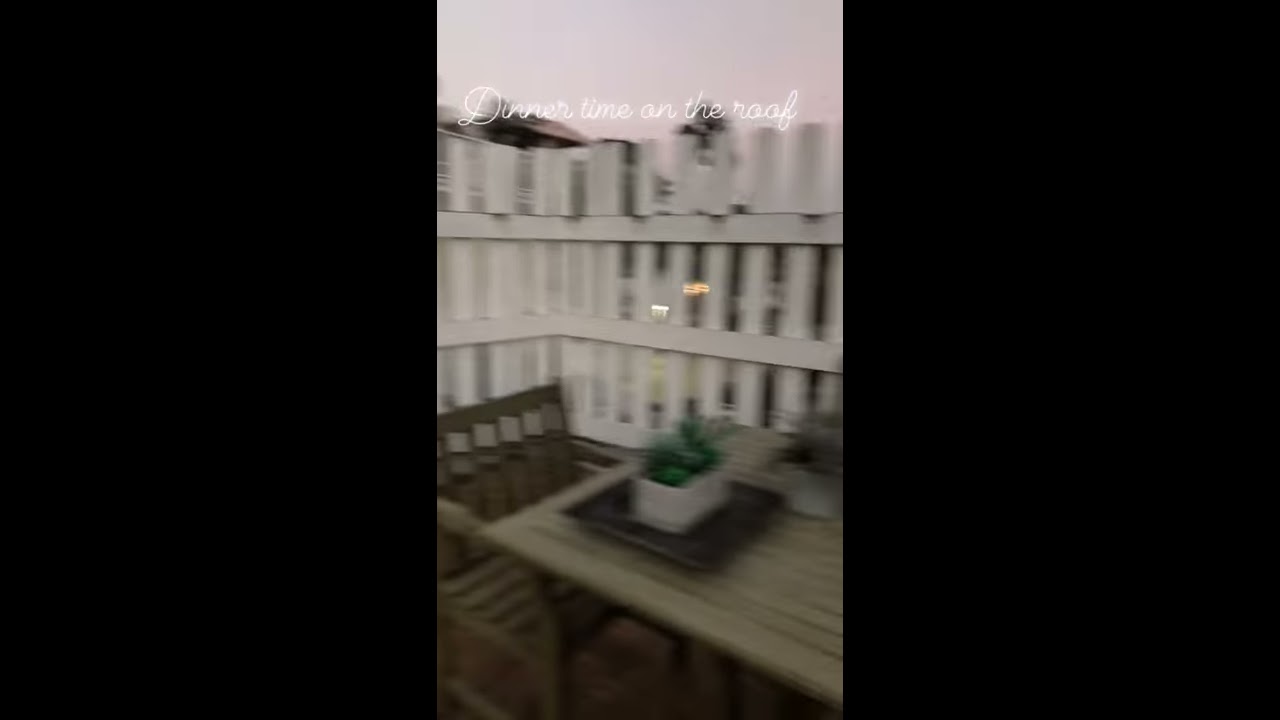This image captures a cozy, albeit blurry, outdoor dining scene labeled "Dinner on the Roof" in elegant white cursive text. It appears to be set on a patio or rooftop, enclosed by a tall, slatted white fence approximately eight feet high. The centerpiece is a rustic wooden table with a light brown hue, slightly warped to give it a vintage charm. Accompanying the table are two wooden slatted chairs, similarly light brown in color. Placed centrally on the table is a brown tray holding a white pot with a vibrant green plant, alongside another white pot containing a green plant. The background features an overcast sky tinged with hues of pink and light filtering gently through the gaps in the fence.